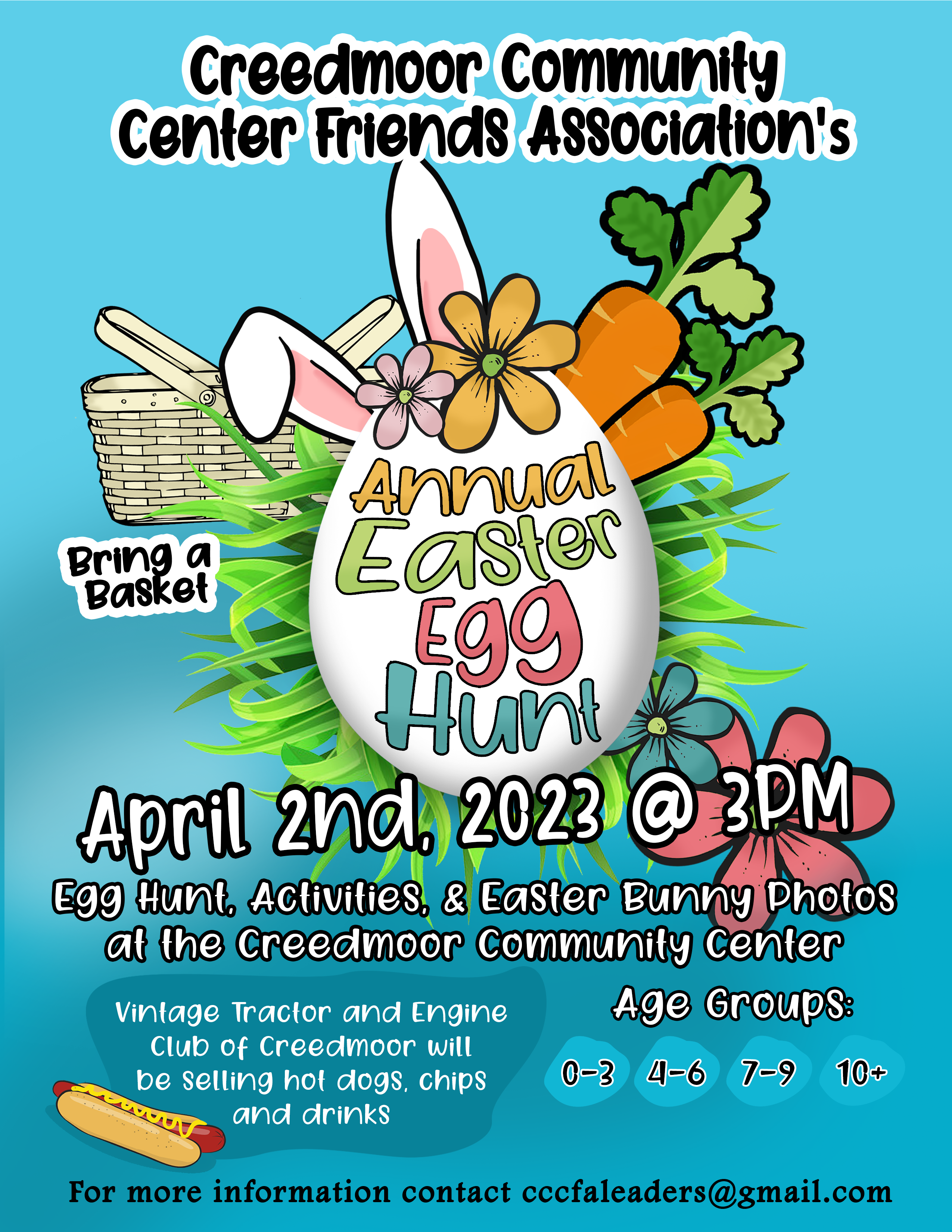This poster, designed with a light turquoise blue background, announces the Creedmoor Community Center Friends Associations’ Annual Easter Egg Hunt. The heading at the top is in black stylized print with white borders, spelling out "Creedmoor Community Center Friends Associations," with an unusual apostrophe after "Associations." 

Central to the poster is a large, stylized Easter egg adorned with bunny ears and surrounded by various decorations, including carrots with green stems, and flowers in pink, yellow, and violet hues. The text on the egg itself is vivid and colorful: "Annual" in yellow, "Easter" in green, "Egg" in pink, and "Hunt" in a darker greenish-blue.

To the left of the egg, a brown wicker basket with handles and green grass poking out is illustrated, with the caption “Bring a Basket” beneath it. Directly underneath the egg, in crisp white text, are the event details: “April 2nd, 2023 at 3 PM” followed by “Egg Hunt, Activities, & Easter Bunny Photos at the Creedmoor Community Center.” 

The age groups for the egg hunt are clearly listed: 0-3, 4-6, 7-9, and 10+. Additionally, the Vintage Tractor and Engine Club of Creedmoor will be present, selling hot dogs, chips, and drinks, indicated in white text beside a depiction of a hot dog with mustard at the bottom left corner. 

For further information, attendees are directed to contact “CCCFAleaders@gmail.com,” written in black type at the bottom of the poster. The lack of a physical address for the Creedmoor Community Center suggests it’s a well-known local venue.